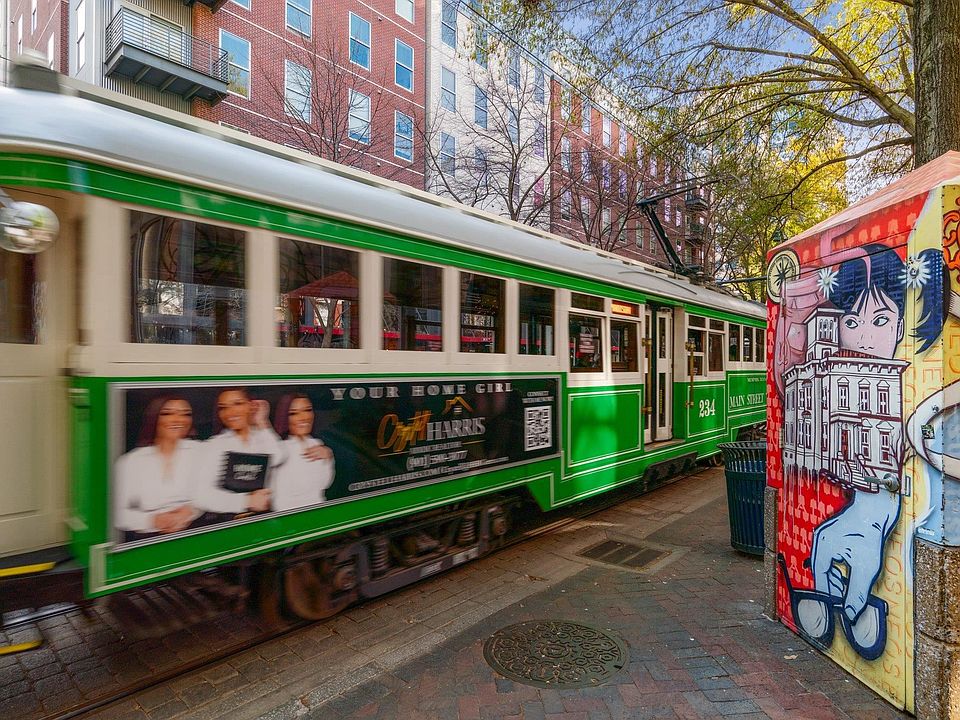In the daytime outdoor photograph, a vibrant green and white subway train with a silver or light brown roof rolls above ground through a cityscape. An advertisement on the train, promoting real estate, features the slogan “Your Home Girl” and includes the name “Harris” alongside an image of three women holding a black book. The ad functions like a mobile billboard. The train bears the markings “Main Street” and the number “234”. The scene is set against the backdrop of multi-story apartment buildings, constructed from both red and off-white bricks, with numerous windows and a noticeable black balcony on one. Overhead, electrical lines power the train, while lush green leafy trees extend their branches into the frame, hinting at a transitional season, likely spring or early fall.

The street below is paved with cobblestones and features various urban elements, such as a manhole cover, drainage grate, and bright red and black brick sidewalks. To the photograph’s right, a detailed mural painted on a wall adjacent to a tree shows an Asian girl with pigtails adorned with daisies, a hand holding a pair of glasses, and a building in white with red accents. The mural adds an abstract, artistic touch to the urban environment. No people are present, and the image is wider than it is tall, capturing a panoramic slice of the city's vibrant street life.